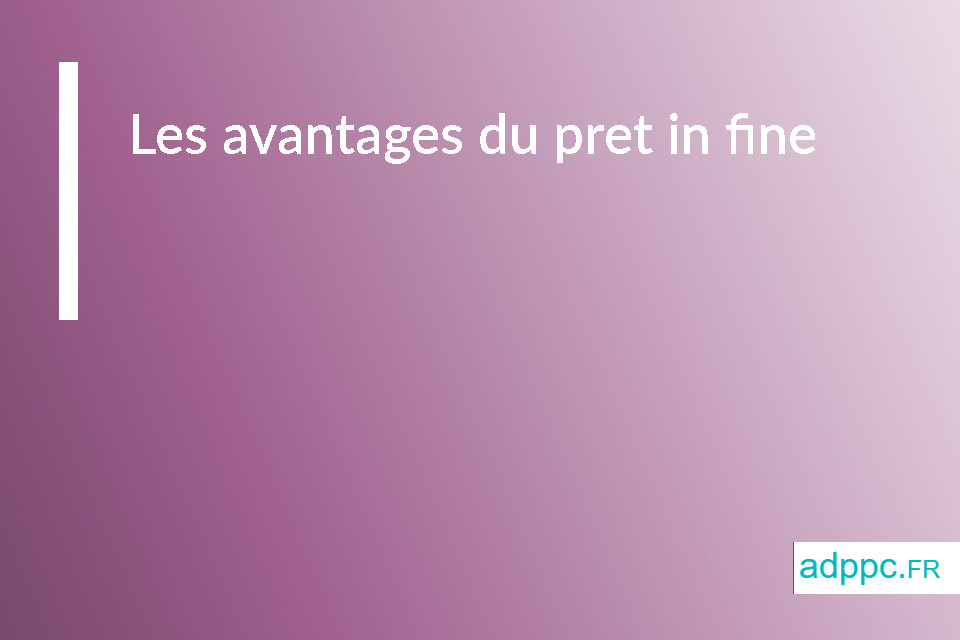The image appears to be a digital advertisement or a PowerPoint slide with a gradient background transitioning from medium purple on the left to a very light pink on the right. A white vertical bar is present, taking up about 5-10% of the left side and running down to around 50% of the image height, indented slightly from the left edge. At the very top of the image, in a language resembling French, the title reads "Les Avantages du Pret en Fin." In the lower right corner, inside a white box with teal text, is the website address "adppc.fr." The design is simplistic and contains no actual objects, suggesting it is meant for digital presentation or as a web graphic.